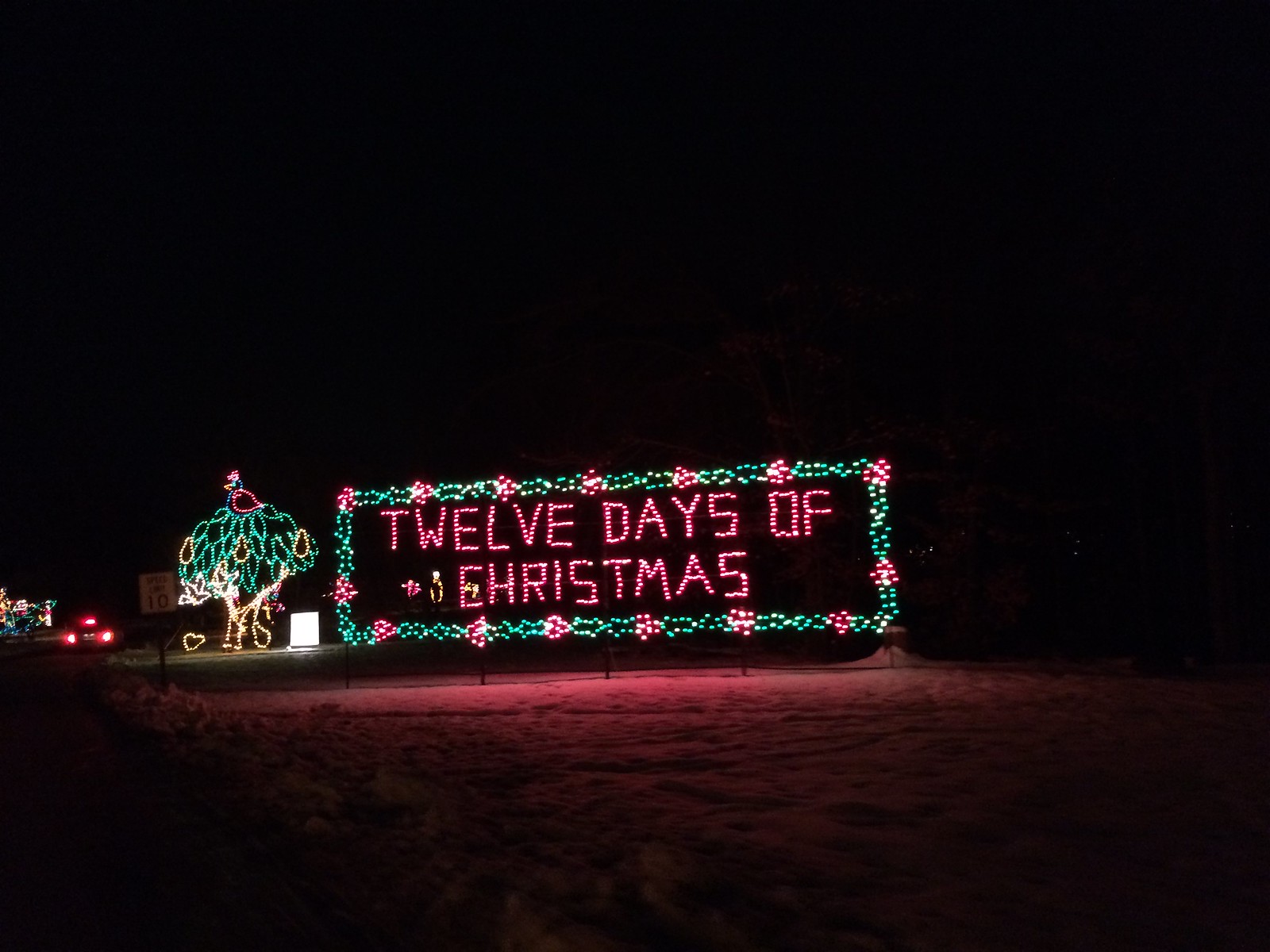This photograph, taken at night, captures an enchanting Christmas light display set against a dark backdrop, likely situated beside a snow-covered roadway. At the center of the display is a brilliantly decorated tree adorned with green, white, and red lights, topped with an outline resembling a parrot, imparting a tropical flair. Adjacent to the tree is an illuminated sign reading "12 Days of Christmas." The sign is crafted in red lighting and bordered with alternating green and red lights that emulate evergreen branches and poinsettia flowers, creating a festive chain-like effect. Adding to the scene's festive ambiance is a nearby billboard adorned with lights fashioned to resemble holly leaves and berries, also bearing the "12 Days of Christmas" message. Further along, another light installation depicts a partridge in a pear tree, intricately designed with Christmas lights. The scene appears devoid of people and is likely located in an empty lot or in front of a business, adding to its tranquil charm.